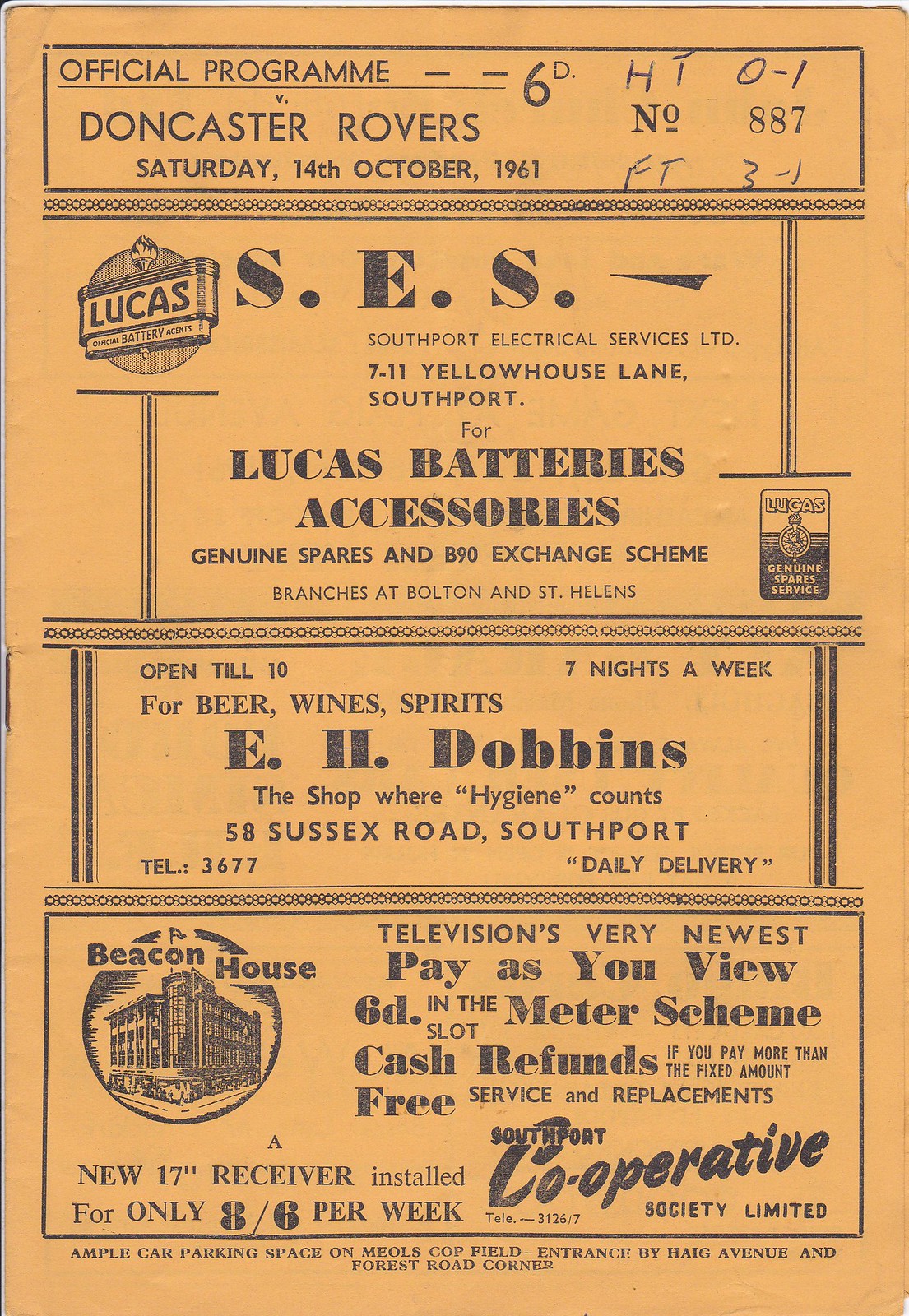This is a worn and faded game day program for a soccer match between Southport and Doncaster Rovers, dating back to Saturday, October 14th, 1961. The cover is a yellowish-gold color with all lettering in black. At the top, it reads "Official Program 6D v. Doncaster Rovers, Saturday, 14th, October 1961, Issue Number 887." Handwriting on the top notes "HT 0-1" and "FT 3-1." Below the title, the first advertisement is for "SES, Southport Electrical Service Limited, 711 Yellow House Lane, Southport," detailing services for "Lucas Batteries Accessories, Genuine Spares, and B90 Exchange Scheme." Branches are also listed at Bolton and St. Helens. Next, there's an advertisement for "EH Dobbins, the shop where hygiene counts," located at "58 Sussex Road, Southport," which is open until 10 PM daily, offering beer, wine, and spirits with telephone contact 3677 and daily delivery. The third advertisement for "Beacon House" features an illustration of a building in the left corner, promoting "Television's very finest pay as you view, 6D in the slot meter scheme, offering cash refunds if you pay more than the fixed amount, free service, and replacements," provided by "Southport Cooperative Society Limited."